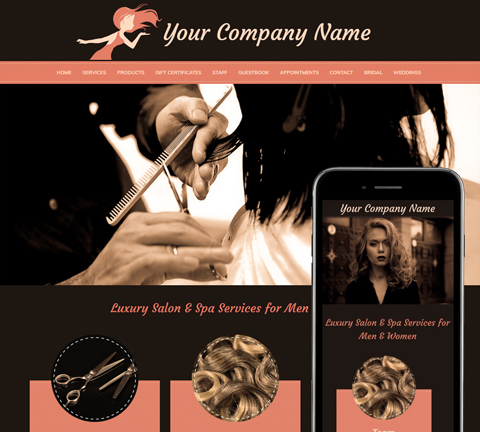The image showcases a square website template designed for a salon. At the top, there is a sleek black header bar featuring the text "Your Company Name" and to the left, an illustration of a woman with flowing hair, appearing to blow a kiss towards the company name. Directly beneath this is a navigation bar in a light red hue, listing menu options such as Home, Services, Products, Gift Certificates, Staff, Guest Book, Appointments, Contact, Special, and Weddings. 

The main section displays a monochrome image with red accents, depicting a hairdresser’s close-up hands cutting the ends of long hair with scissors and a comb. The subject’s shoulders are draped with a protective cloth, creating a sophisticated, almost black-and-white atmosphere. Below this image, the banner reads, "Luxury Salon and Spa Services for Men."

Three service icon sections appear beneath the main image, highlighting illustrations such as a pair of scissors and strands of hair. Additionally, the bottom right corner features a mock-up of the mobile version of the website, presenting a similar layout but optimized for a phone. In the mobile version, "Your Company Name" is followed by a fashion-forward image of a woman with stylish hair. The tagline below reads, "Luxury Salon and Spa Services for Men and Women," completing the inclusive appeal of the template. The website’s color scheme predominantly uses black and a peachy red, enhancing the elegant and professional vibe.